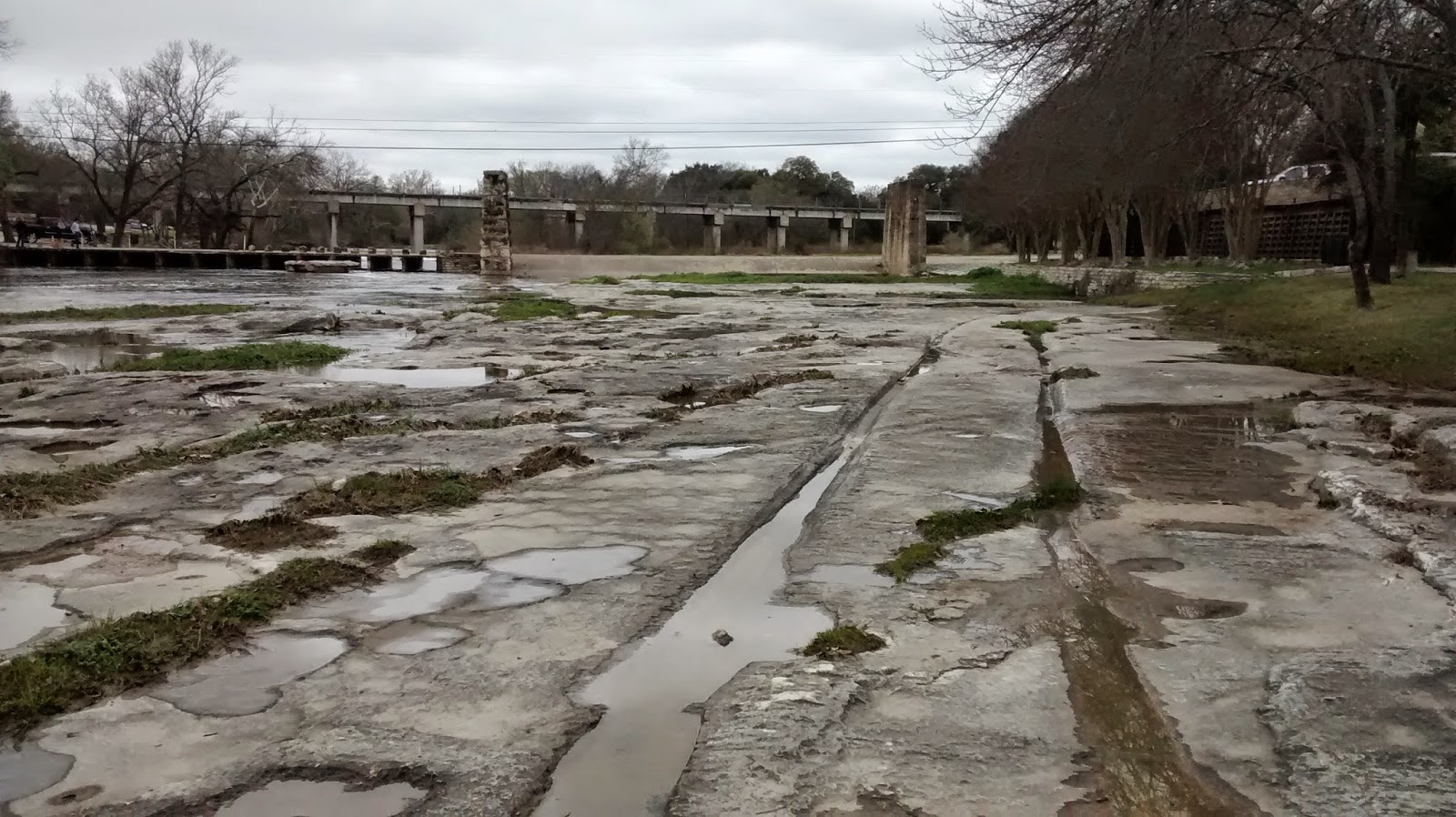The image depicts a large, abandoned concrete area that appears to be part of an old parking lot. The cement is heavily weathered, riddled with numerous cracks and potholes, with grass and moss growing through them, indicating neglect and disrepair. Rainwater has collected in the cracks, creating small puddles throughout the scene. On the left side, there's a small stream or river visible, spanned by a modest bridge, while a taller, older bridge, possibly for trains, stands in the background supported by stone pillars. The horizon is lined with trees, many of which are bare, suggesting a wintry season. The sky above is overcast and gray, shrouded in clouds. On the right side, there's a brown building partially obscured by tall trees, with patches of dead, brown grass nearby. Overall, the scene conveys a sense of abandonment and decay, enhanced by the dreary weather.